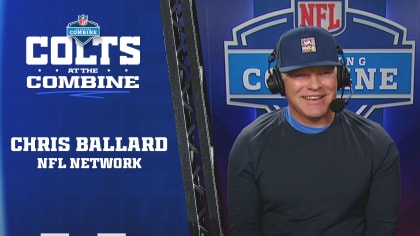This landscape photograph captures a lively moment with Chris Ballard, the host from the NFL Network, at the NFL Combine. Positioned on the right side of the image, Ballard is smiling warmly towards the camera, embodying a sense of enthusiasm and professionalism. He is wearing a navy blue baseball cap, a dark blue long-sleeve shirt layered with a brighter blue shirt underneath, and a black headset with a large microphone. His eyes are slightly squinted, yet his smile is evident, suggesting he is engaged in broadcasting. On the left side of the image, a graphic reads "Colts at the Combine" in white text and directly below it, "Chris Ballard NFL Network." The backdrop features a blue theme with hints of text, including an NFL logo in red and indistinct combine-related lettering, reinforcing the context of the NFL scouting event.